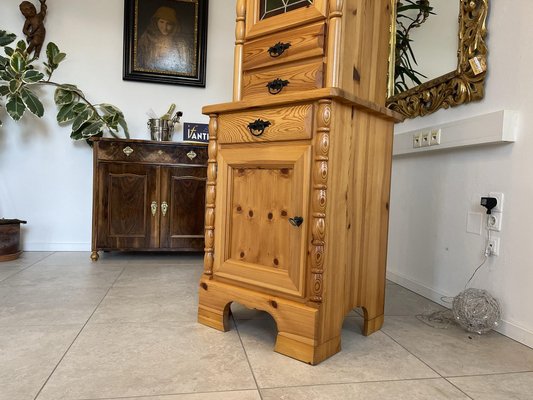In the living room, a light-colored wooden cabinet with prominent dark knots sits on large gray ceramic tiles. The cabinet features a square door with four dark knots in the middle and one in each corner, accented with black handles. Above the door is a drawer on the left, also with a black handle. The top section of the cabinet has two rectangular drawers with black handles, and above them is another door featuring a glass window. 

To the left of this centerpiece, another standalone dark wooden cabinet, marked with yellow stains and gold handles, is positioned against the wall. It has a wide-handled drawer at the top. Above this cabinet, a portrait in a black frame hangs on the wall, with white light reflecting off its surface. Adjacent to the portrait on the left, large dark green leaves emerge from a branch.

The right side of the room shows a white-painted 2x4 mounted on the wall, with three light-colored wire outlets. Near the bottom, a bundle of gray wire and an electric socket with attached LED wires can be seen. The room’s walls are white, enhancing the contrasting details, and creating a balanced yet diverse aesthetic.